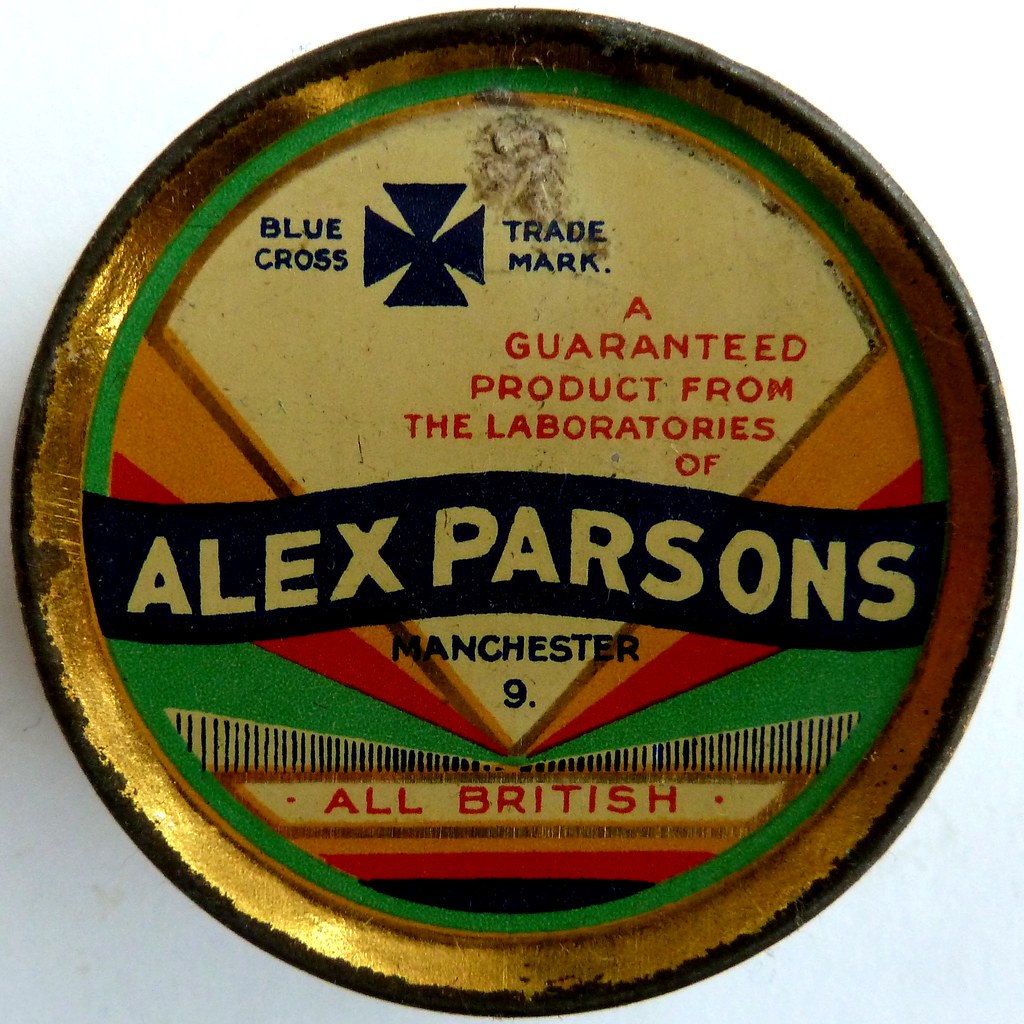This is a detailed photograph of a round metal lid, embellished with a colorful array of designs and text. The central focus is a blue banner across the beige background that prominently displays the name "Alex Parsons" in black text. Encircling the lid is a gold rim, although some parts are tarnished and peeling. The top of the lid features the words "Blue Cross Trademark" in blue print, accompanied by a blue cross symbol. Below this, in flowing black text, it reads "Alex Parsons" and "Manchester Nine" in blue print, followed by "All British" in red print. Further down, in red print, it states, "a guaranteed product from the laboratories of Alex Parsons." The backdrop of the lid is a vivid mix of green, red, and yellow, with decorative fan shapes and thick lines in gold, red, blue, and white adding to the visual intricacy. The myriad of colors and patterns, combined with the detailed, multi-colored text in blue, black, and red, make the lid both eye-catching and enigmatic, leaving the actual contents of the jar or can a mystery.